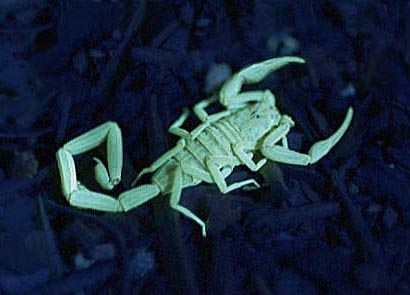The image features a pale green scorpion, prominently positioned in the center against a dark, almost nighttime background that combines deep blues and blacks, resembling dark mulch or stones. The scorpion, which could be a 3D model or even a 3D-printed figure, exudes an eerie glow that gives it a glow-in-the-dark appearance. Its segmented tail curves gracefully towards the bottom left of the image, composed of six distinct sections reminiscent of connected pasta noodles, with a menacing stinger at the tip. Positioned with precision, its two prominent pincers extend towards the top right, ready to strike. The scorpion's body is flanked by three small legs on each side, showcasing its intricate anatomy. The creature's back displays noticeable banding, adding to its realistic and detailed depiction. This striking composition could be mistaken for an advertisement, despite the absence of any text, focusing solely on the captivating, luminous scorpion against the dark, textured backdrop.